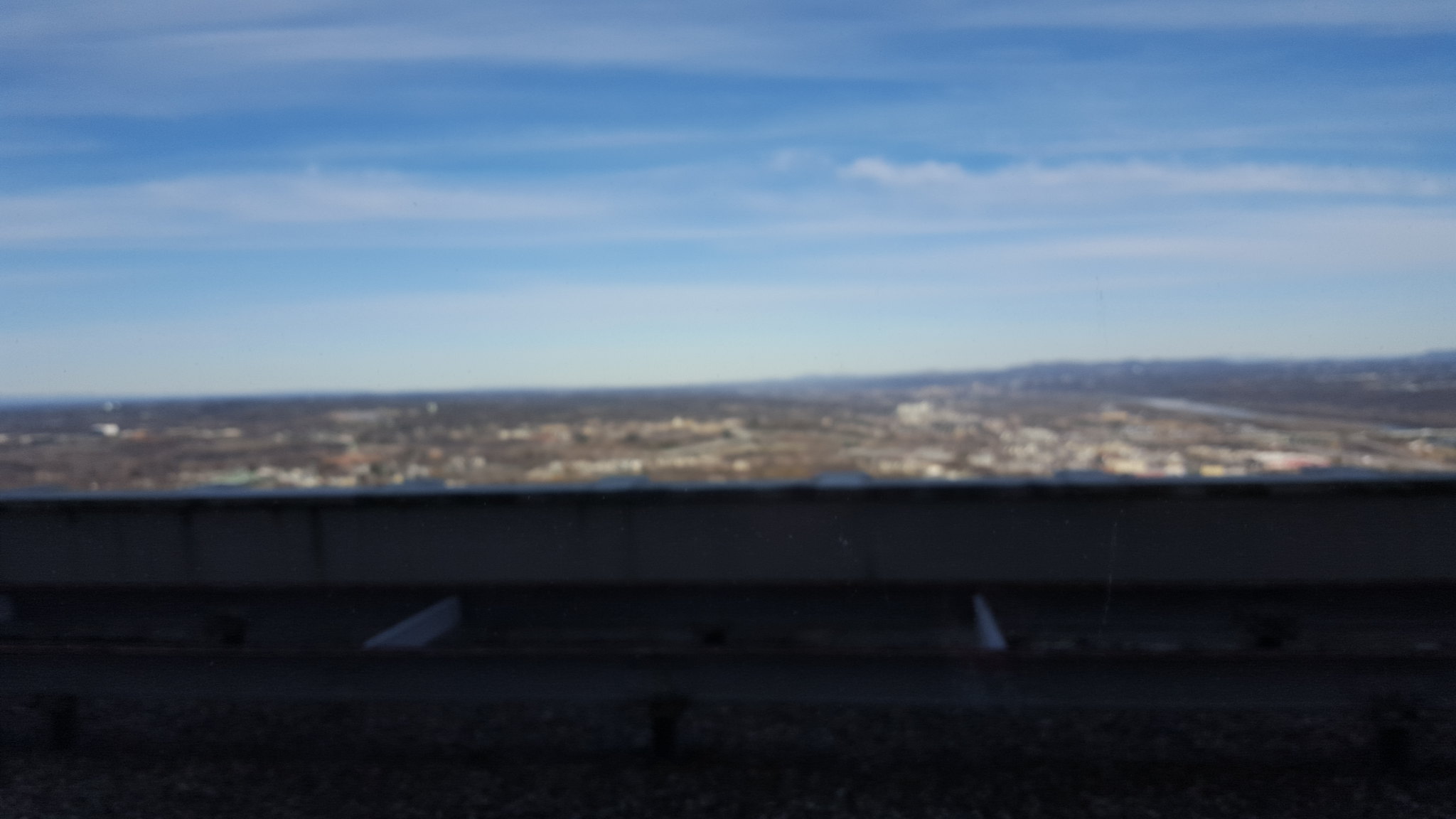A blurry photograph captures a rooftop scene with a flat surface covered in fine gravel. The photographer appears to be standing on this rooftop. Prominent in the foreground is a horizontal dark gray bar, accompanied by several vertical bars. A slightly elevated gray wall is visible just beyond these bars. In the background, although the details are obscured, a light blue sky can be seen along with hints of blue water and blurred images of white and brown buildings. There is an indistinct, large brown streak on the right side of the image, possibly positioned above a river, adding to the enigmatic nature of the scene.